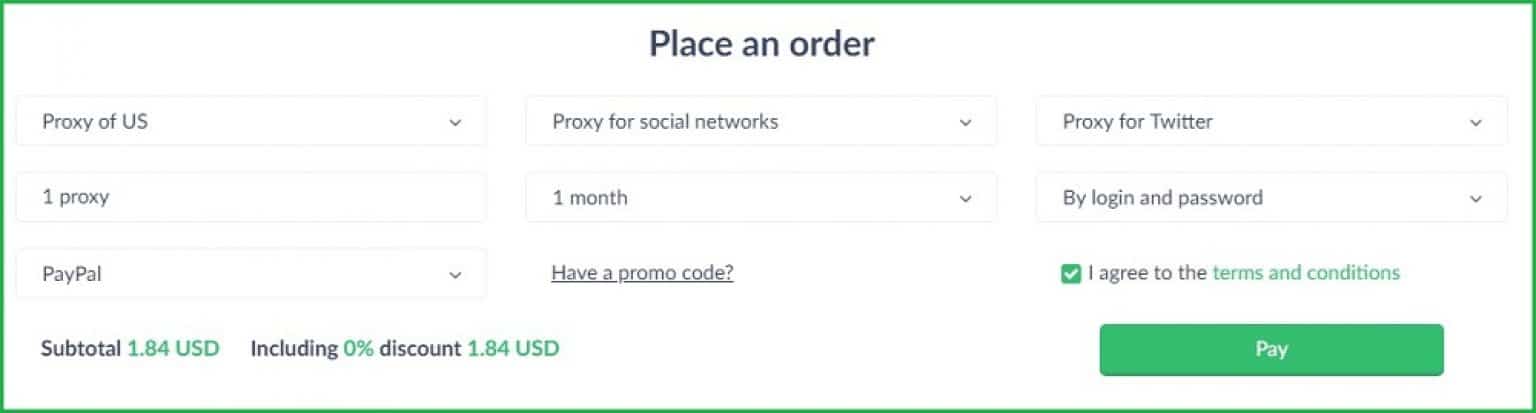**Detailed Caption:**

A web page interface for placing an order, prominently featuring a green border enclosing the entire section. The top part of the page displays the text "Place an Order." Within the bordered area, there are seven distinct white boxes arranged systematically. 

- The first box includes a label "Proxy Type" with an accompanying drop-down menu for selection.
- The second box is labeled "Quantity" and specifies "1 Proxy."
- The third box reads "Payment Method" and is equipped with a PayPal drop-down menu.

Adjacent to these, another set of options is presented:
- The first box in this column is labeled "Proxy for Social Networks" with a drop-down menu.
- Below it, a box labeled "Duration" includes a drop-down menu for selecting "One Month."
- Beneath this, a prompt labeled "Have a Promo Code" with an entry field follows.
- Next, there is a section for "Proxy for Twitter" specified by login and password fields.

Below these options is a checkbox labeled "I agree to the terms and conditions," which is marked with a green check. Directly beneath this agreement section, a prominent green payment button is visible. 

In the bottom right corner, the subtotal is clearly indicated as $1.84 USD, including a 0% discount. This amount represents the total cost of the order. 

Overall, the page is intended for ordering proxy services with various customization options, clear payment instructions, and terms agreement features.